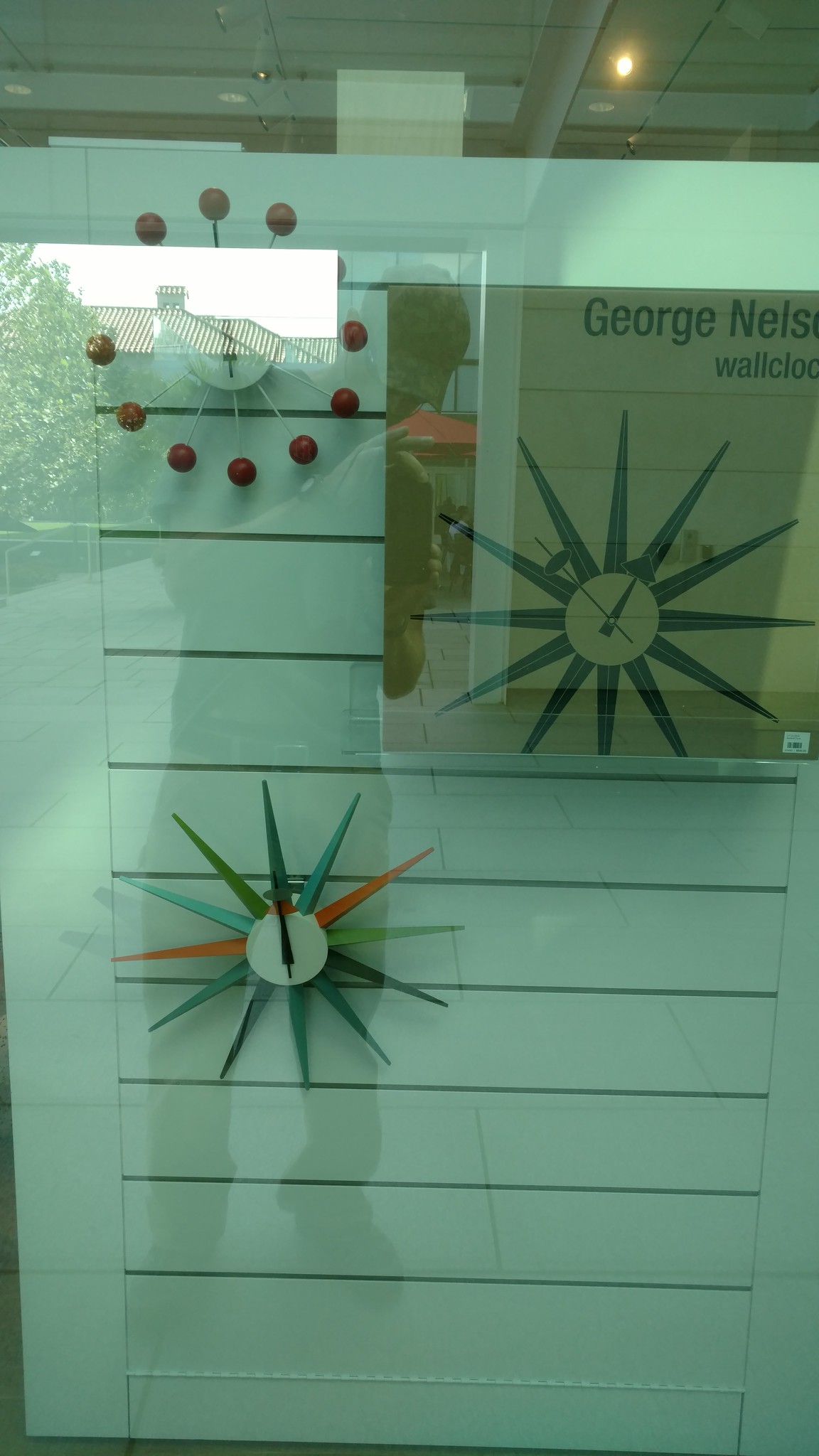This photograph captures a reflective storefront window with the full-bodied reflection of a young man, wearing a baseball cap, long pants, and a short-sleeved shirt, holding a cell phone vertically to take the picture. The glass has a greenish tint, highlighting two distinct modern wall clocks in the display. One clock features a colorful starburst pattern with spindly arms ending in green, blue, and orange triangles, a plain white clock face, and black hands indicating 12 o'clock. The second clock, positioned above the first, showcases a burst design with small white spindles tipped with red bulbs and a central white clock face with black hands. A brown square sign in the top right of the display reads "George Nelson wall clocks" in black text. The scene outside also includes the faint reflection of a building and a tree, adding depth to the composition.